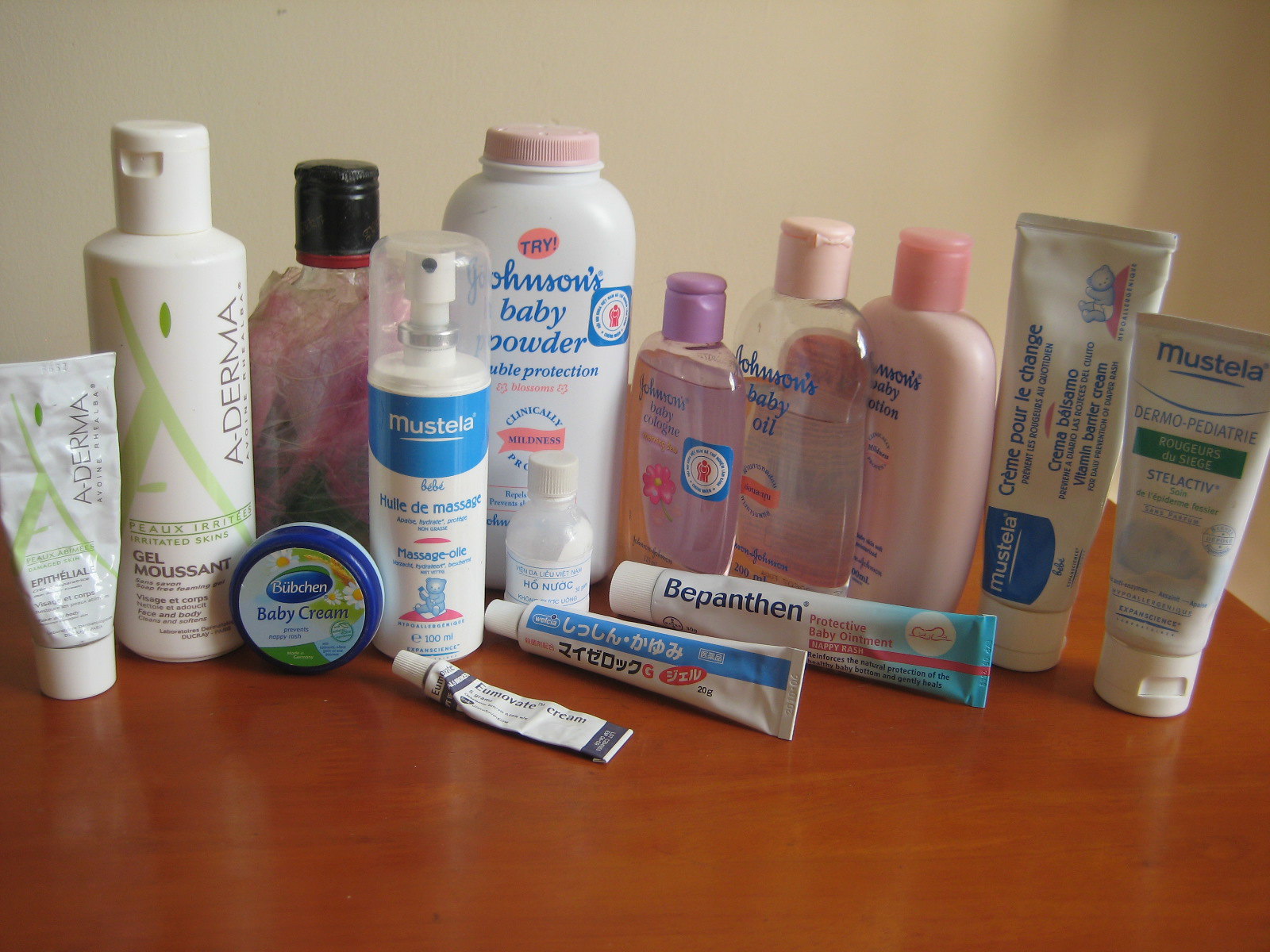This detailed photograph showcases a variety of baby care products neatly arranged on a wooden surface against an off-white background. Each item offers a glimpse into the meticulous care that goes into choosing the best for a baby's needs:

1. **A-DERMA Epithelial Cream:** A white metal tube adorned with green designs. The primary text reads "ADERMA" and "EPITHELIAL" in black, although the finer green and black text are not discernible.
   
2. **A-DERMA Gel Moussant:** A white bottle, echoing the design of the cream tube, with the name clearly displayed. The label includes "GEL MOUSTANT" and "IRRITATED SKINS" in green text. It has a practical flip-top cap.

3. **Baby Cream Tin:** A small, round tin featuring a sky blue lid with illustrations of green grass and white daisies with yellow centers. The rim of the lid is also blue.

4. **Decorative Bottle:** A clear bottle wrapped in pink and partially green gauzy fabric, capped with a black metal lid trimmed with red. It lacks any visible text.

5. **Mustela Massage Oil:** This white bottle features "MUSTELA" in white on a blue label. It is capped with a clear lid, revealing an aerosol or pump dispenser beneath. The bottle showcases French and English text, "HUILE DE MASSAGE" and "MASSAGE OIL," alongside an image of a teddy bear seated on a pink surface.

6. **Johnson's Baby Powder:** A larger white plastic container with a pink twist lid. The label contains a pink oval with "TRY" in blue and "Johnson's Baby Powder" below it. Additional details include "PROTECTION," "BLOSSOMS," and "CLINICALLY MILDNESS."

7. **Small Bottle with Foreign Text:** This short, clear bottle with a white lid has an illegible label except for the letters "H-O-N-U-O-C."

8. **Eumovate Cream:** A nearly depleted small metal tube with gray trim and text reading "EUMOVATE CREAM."

9. **Asian-Labeled Cream Tube:** A metal tube with a light blue stripe and a mix of Asian characters and pink accents.

10. **Bepanthen Protective Baby Ointment:** A tube featuring blue and pink text, including "BEPANTHEN" and details about its protective and healing properties for baby's skin.

11. **Johnson's Baby Cologne:** A clear bottle with a lavender lid, labeled in blue. It features a pink flower and a blue sticker with a red image.

12. **Johnson's Baby Oil:** A clear bottle with "Johnson's Baby Oil" in blue text, capped with a pale pink lid.

13. **Johnson's Baby Lotion:** A pale pink bottle with a darker pink lid.

14. **Mustela Vitamin Barrier Cream:** A white tube with distinct blue and pink labels. It is marked as a diaper rash protection cream with French and English instructions.

15. **Mustela Stelactiv Cream:** Another white tube with blue and green labeling, featuring the terms "DERMOPEDIATRIE" and "STELACTIV."

Each of these carefully chosen items reflects a dedication to baby care, providing a visual narrative of products ranging from essential creams to thoughtful colognes, all designed to ensure the well-being of infants.